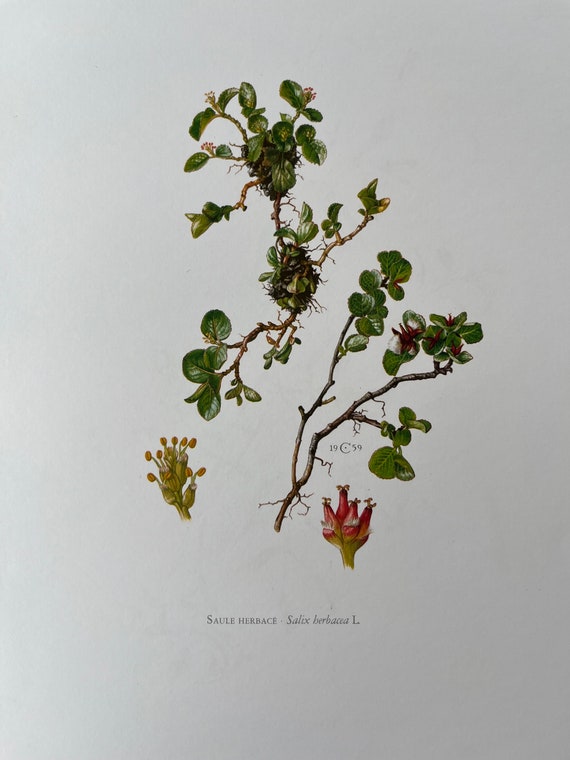This detailed botanical illustration, likely dating from 1939, features a species of willow, identified by the inscription "Salix," possibly from the family Salicaceae. The illustration, rendered in old-fashioned watercolor on a white background, depicts a low-growing, shrubby ground cover plant with rounded, somewhat waxy green leaves. The branches bear tiny flower buds that are yellow with small round bulbs. Highlighted on the illustration are close-ups of the plant's delicate red flowers, which have tiny yellow pollen grains at their tips, providing a clearer view of these otherwise insignificant blooms. The detailed close-ups offer an enhanced perspective, ensuring the intricate features of the buds and flowers are distinctly visible.